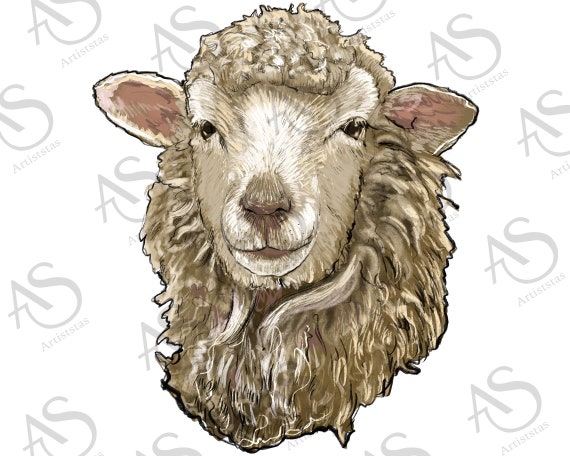This square image features a detailed digital artwork of a sheep's head, combining elements of both cartoonish and photorealistic styles. The sheep has a predominantly brown face with shades of white and pink interspersed, particularly between its eyes, around its mouth, and at the inside of its ears. The ears, which point outward, have a pinkish-brown interior bordered by tan. The sheep’s closed-mouth expression gives an impression of a subtle smile. Its wool is textured with bumpy curls, showing a mixture of brown and white hues. The headshot, extending just below the neck area, displays shading in darker and lighter browns, emphasizing the texture of the wool.

This artwork is set against a plain white background, free of any borders. Diagonally printed across the image are the letters "A-S," with the S being larger and curling into the center of the A, forming a logo. Beneath this logo, the word "Artistas" is printed in gray. The logo and the word are repeated across the background and the sheep’s head like a watermark, adding a layered texture to the overall image.